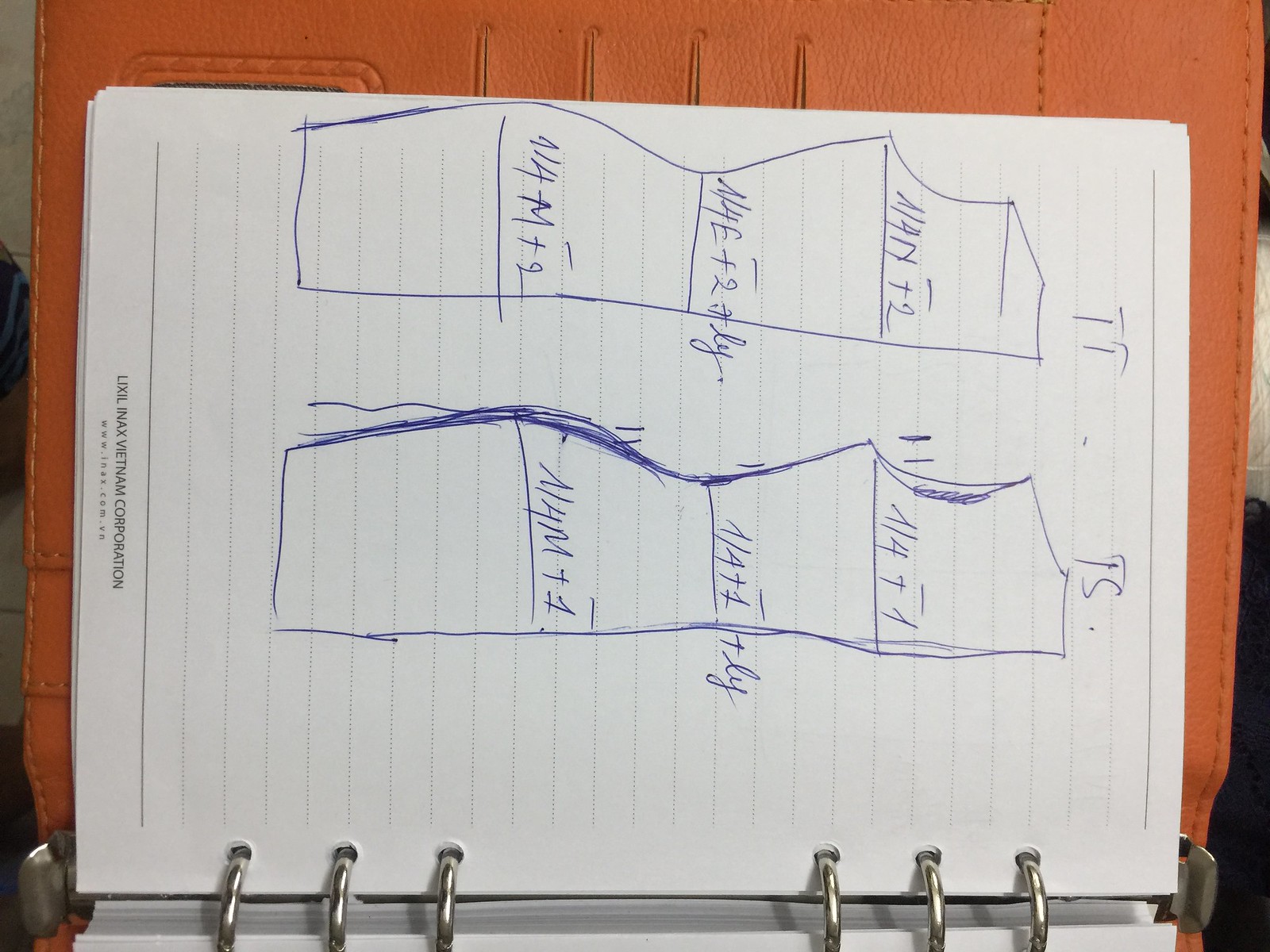The image depicts a white sheet of paper adorned with intricate blue sketches, likely representing various fabric patterns or dress designs. The paper is oriented flat on a surface, with the designs facing right. On the top of the drawings, distinct labels are visible, including "TT" and "TS." The text annotations include technical notations such as "A for N plus 2," "N for E plus 2," "LY," and "N for M plus 2" alongside additional markings like "1/4 plus 1," "1/4 plus 1 plus LY," and "1/4 M plus 1." An apostrophe is also noted at the top of these sections. At the bottom of the sheet, in black text, the words "LIXIL Vietnam Corporation" are prominently displayed. The paper appears to be part of a larger collection, clipped centrally with metal within what seems to be a diary or binder characterized by an orange cover.